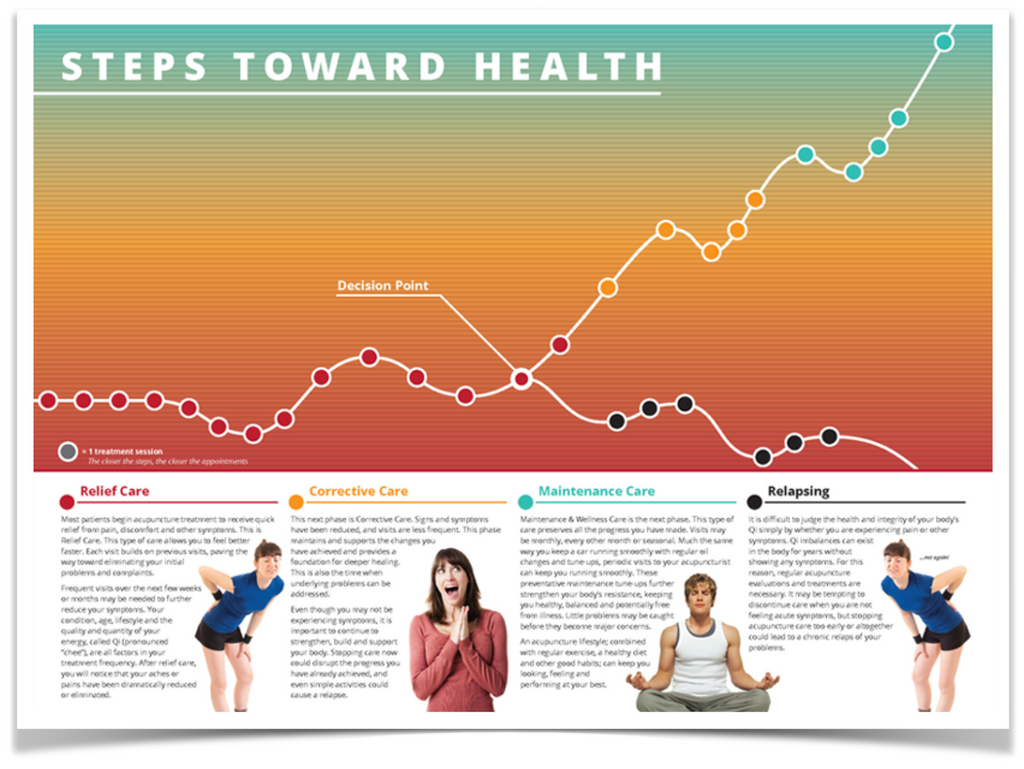This descriptive caption combines all elements and emphasizes common details:

"This poster is about steps towards better health. At the top, white text reads 'Steps Towards Health.' Dominating the center is a rainbow-colored chart which depicts a health progression. The chart starts at the bottom with horizontal red dots, moving upward past a 'Decision Point' marked in white. From the decision point, the chart diverges into two paths: one line ascends, transitioning from red to yellow to blue, while another line curves downward with black dots. The dots are interconnected by white lines.

Below this chart, there are four sections, each with a colored title and an accompanying image. These sections, from left to right, are: 'Relief Care' with a red title and a picture of a woman holding her back in pain, 'Corrective Care' with a yellow title and an image of an excited woman with her hands clasped, 'Maintenance Care' with a blue title and a man in a yoga pose with hands on knees, and 'Relapsing' with a black title and a repeated image of the woman holding her back.

Each section contains paragraphs of text below the images, too small to be read clearly. The background of the poster features a gradient of colors from greenish-blue at the top, fading to orange, yellow, and then red towards the bottom."